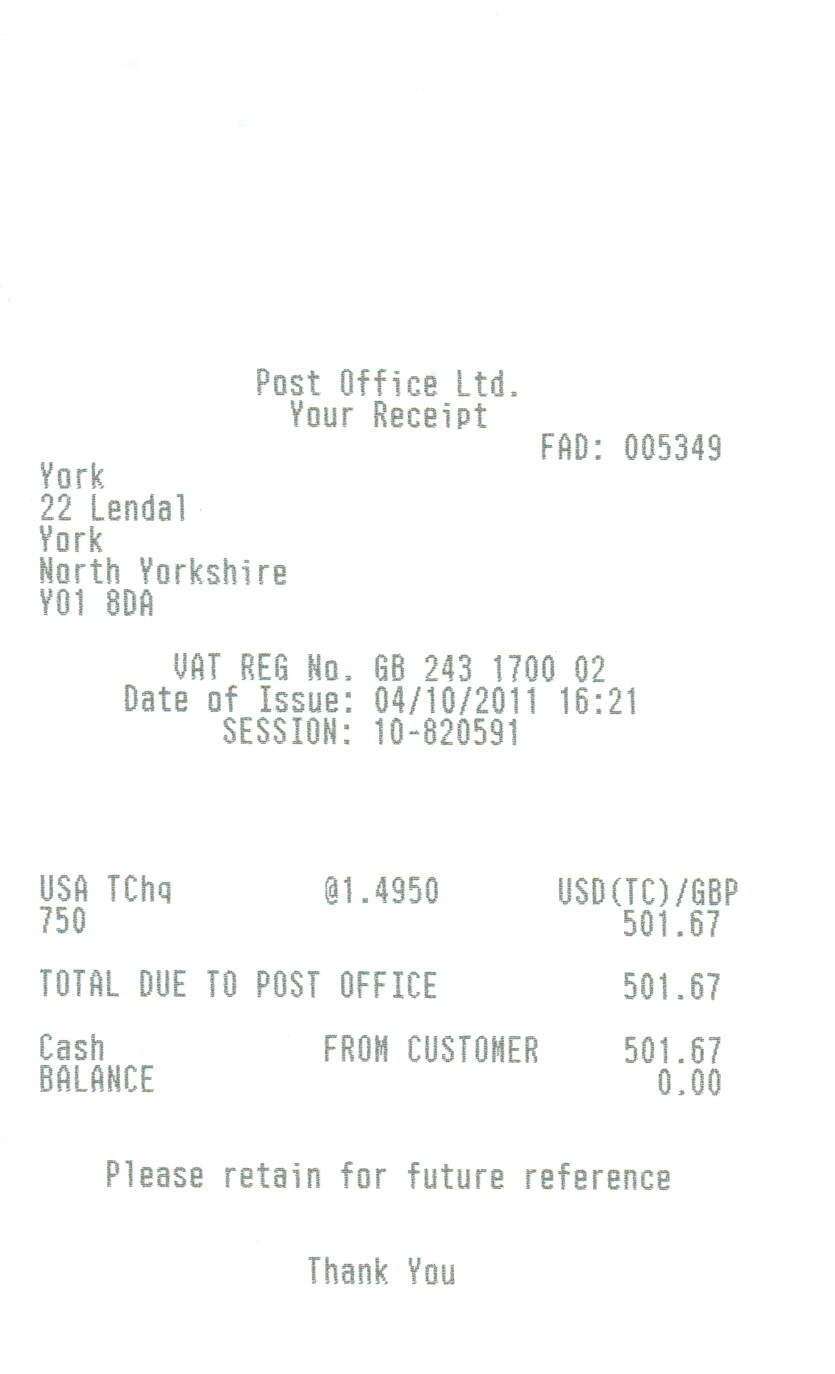The printed image shows a Post Office Limited receipt with the reference number FAD 005349. The receipt was issued in York, specifically at 22 Lendall, York, North Yorkshire Y018DA. The VAT registration number provided is GB 243 1700 02. The date and time of the transaction are October 4, 2011, at 16:21. The session identifier is 10-8205-91. The receipt appears to be for a service possibly denoted by "USA CH Q CH G," although it is partially cut off. The transaction amount recorded is £501.67, and this amount is shown under total paid, total due to the Post Office, and from the customer, indicating the transaction was settled in full in cash. The receipt advises retaining it for future reference and ends with a thank you note from Post Office Limited.